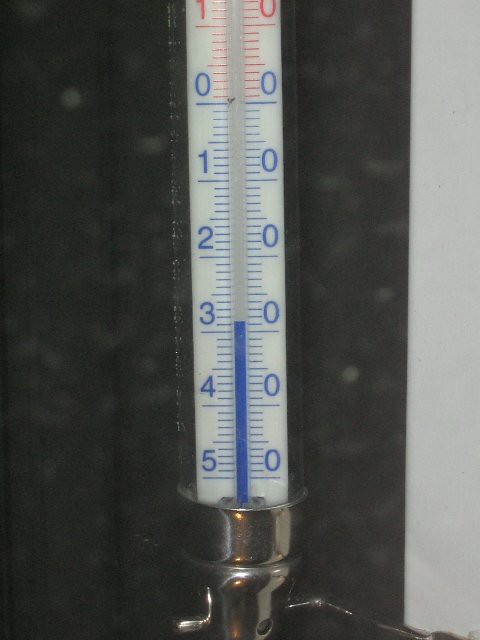This vertically aligned photograph features a contrasting background that is predominantly black, covering approximately three-quarters of the image from left to nearly the far right. The remaining section on the right side presents a stark white background. Central to the image is a thermometer with a sleek silver base. The thermometer's scale is demarcated in blue, with numbers ascending from 0 to 5 from bottom to top. A blue column, indicating the temperature, extends up the thermometer, surpassing the '3' mark. Near the top of the thermometer, part of a red section is visible, with the number '1' on the left and '0' on the right.